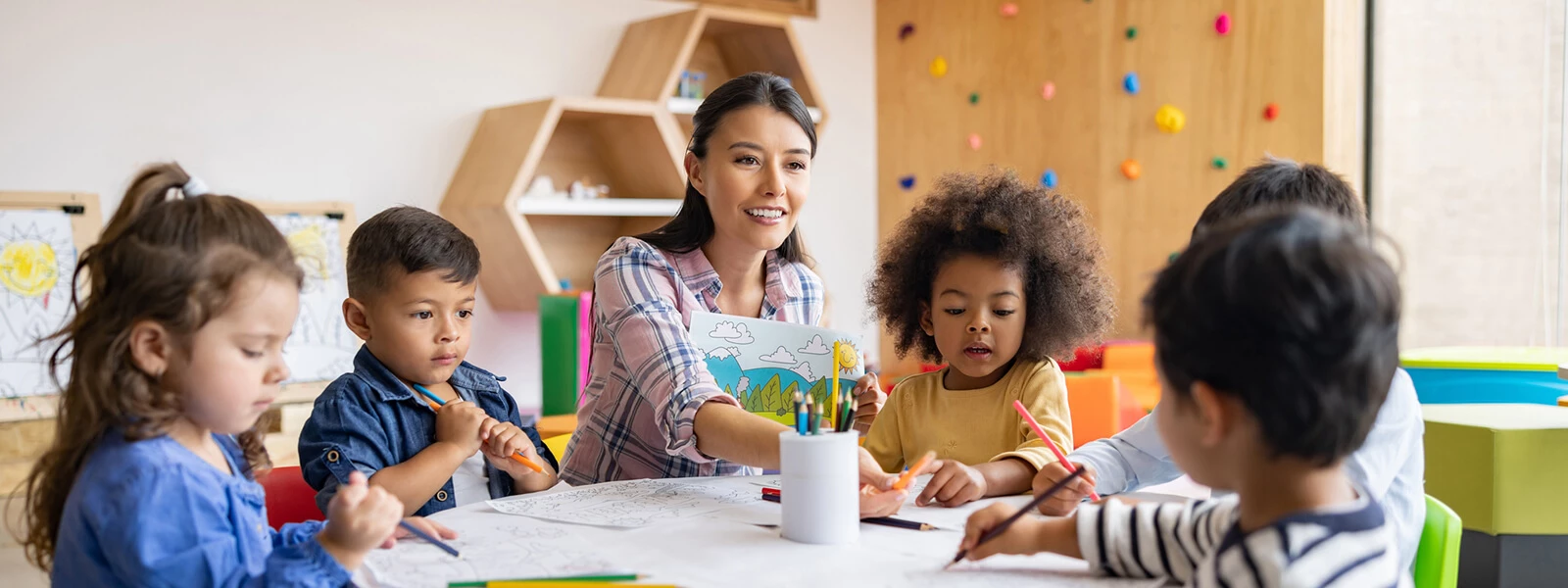This detailed photograph captures a vibrant classroom environment. At the heart of the scene is a white, round table where one adult and five children, appearing to be two girls and three boys, are seated, engrossed in a drawing activity. The adult, likely a teacher, is wearing a pink plaid checked shirt and has her black hair styled half up, half down. She's holding up a playful, cartoony picture of a mountain forest scene with clouds, capturing the children's attention.

The diverse group of children is actively engaged, each holding a colored pencil in an array of colors, including orange, blue, pink, black, and more. The table's centerpiece is a white pot filled with pencils, predominantly in shades of blue, green, and grey. The children's different postures show various levels of focus on their drawing task.

The lively classroom setting is enhanced by a bright and colorful backdrop. Behind the group, there's a climbing wall and hexagon and pentagon-shaped wooden cubbies. Additionally, the wall features posters and an assortment of colorful circular decorations. Various brightly colored stools - green, red, yellow, and orange - add to the room's vibrant atmosphere. The mix of functional and playful elements firmly roots this scene in an educational yet creative and engaging environment.